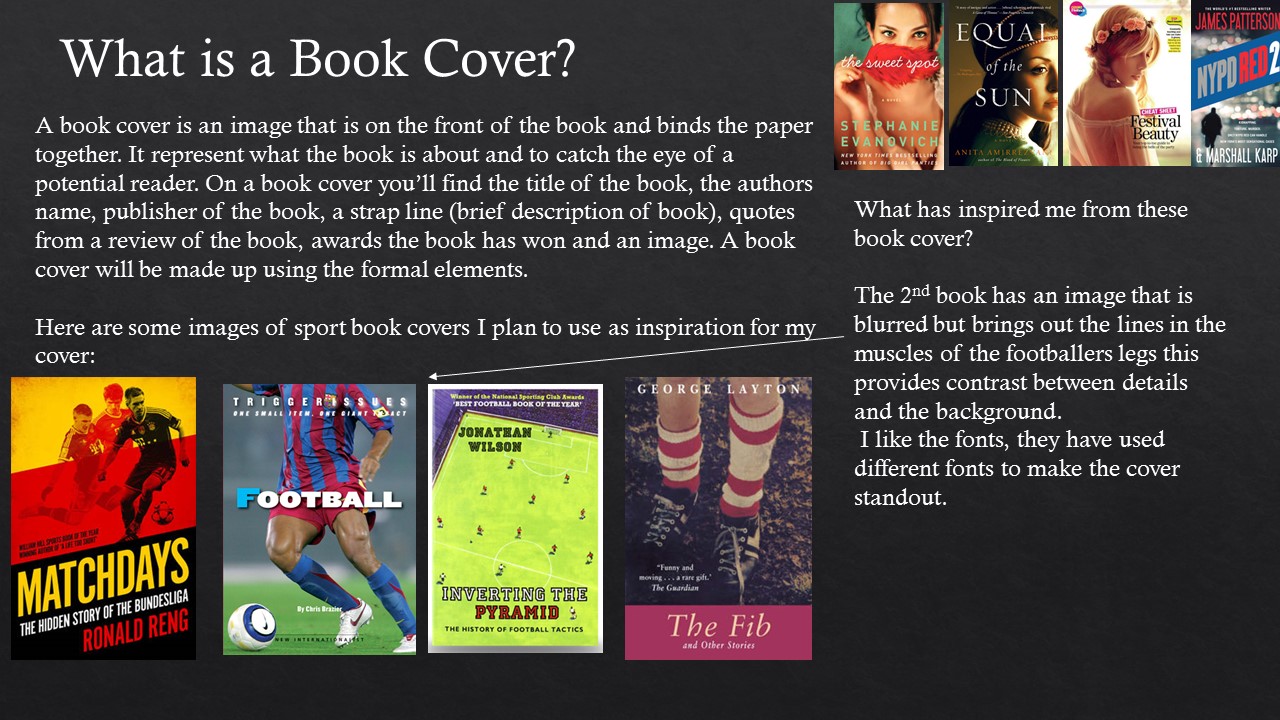The image is a horizontally aligned rectangle featuring a solid black background adorned with both text and small rectangular pictures of book covers. In the upper left-hand corner, white text asks, “What is a book cover?” Below this, there is a detailed left-aligned paragraph explaining that a book cover is an image placed on the front of a book, which binds the paper together. It describes the cover’s role in representing the book’s content and attracting potential readers. The paragraph outlines typical elements found on a book cover, such as the title, author’s name, publisher, strapline, review quotes, awards, and an image. A space separates this from another line stating, “Here are some images of sport book covers I plan to use as inspiration for my cover.”

Beneath this text are four larger rectangular images depicting sports book covers. The covers include: "Match Days" with a red and yellow design, "Football" showcasing a soccer player, "Inverting the Pyramid" featuring a green field with tiny figures, and "The Fib" displaying red and white striped crew socks. 

In the upper right-hand corner of the image, four smaller book covers are displayed. Most of these covers feature female figures, except for the far-right cover, which says "NYPD Red 2." Below these covers, left-aligned, a smaller paragraph reads, “What has inspired me from these book covers?” The text elaborates that the second cover features a blurred image which highlights the lines and muscles of a footballer’s legs, creating contrast with the background. It also mentions an appreciation for the variety of fonts used to make the covers stand out.

Overall, the layout divides the left side of the image for explanatory text and larger book covers, while the right side showcases smaller inspirational covers and additional commentary.